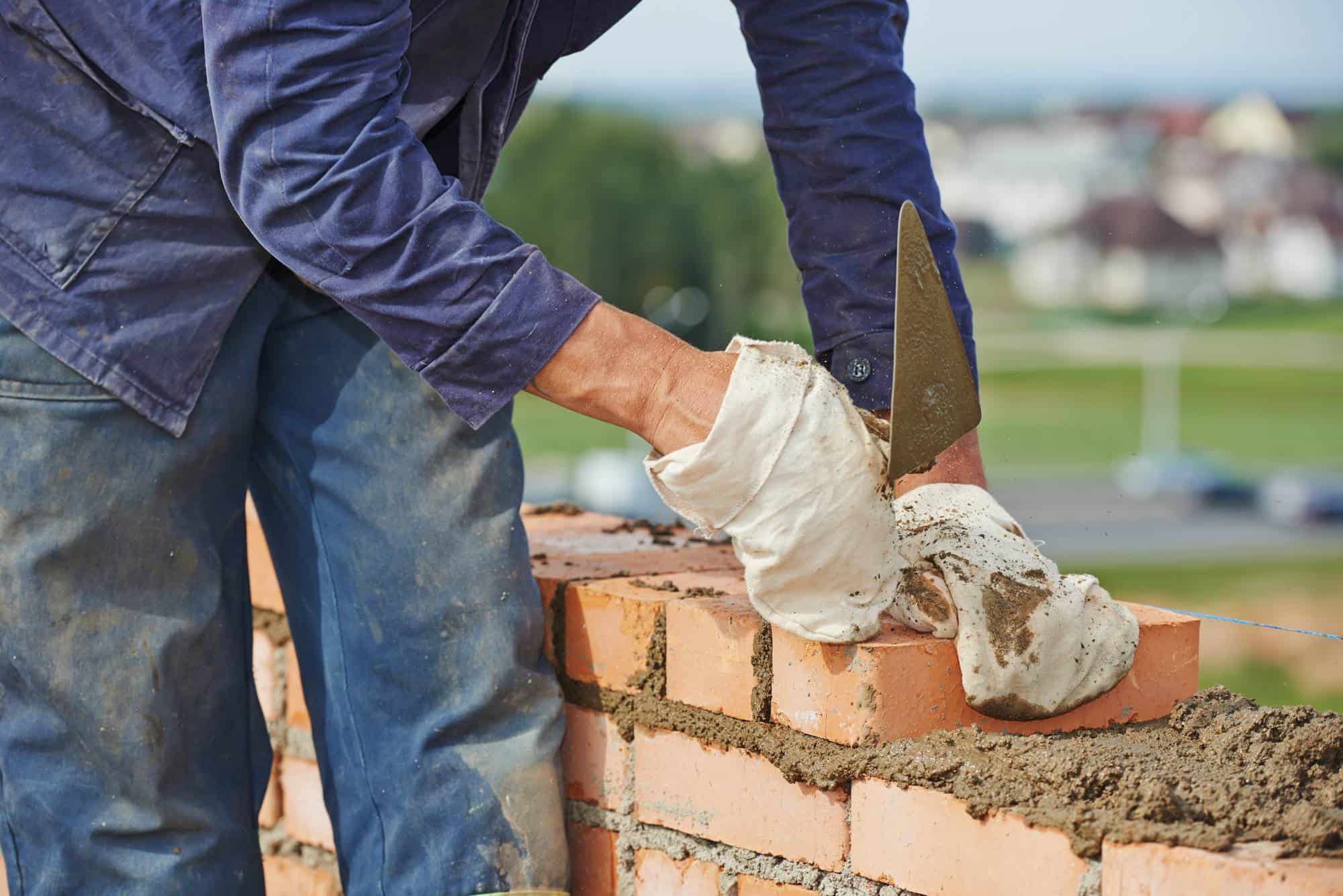In the image, a skilled bricklayer is meticulously aligning bricks to extend a brick fence. The worker, identifiable by their white hands and burlap-like gloves, wields a trowel to spread mortar between the bricks. They are clad in dirty blue jeans and a long-sleeve navy blue jean shirt dotted with pockets. The worker’s gloves and pants bear smudges of the brown, sticky mortar, highlighting the messy nature of bricklaying. The scene is set outdoors, with a blurred background revealing a road, houses, a field, and some trees, giving a sense of the surrounding town without detracting from the detailed focus on the bricklayer’s hands and lower body. The bricks, a pink adobe color, are being laid in a straightforward manner, with the joints left rough and unpolished.